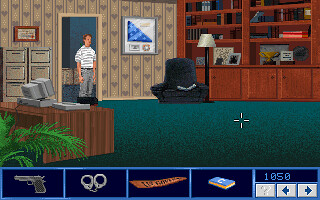This image is a screenshot from a video game depicting a character standing in the doorway of an office room. The room features tan and black wallpaper with beige and brown heart and stripe patterns. The floor is green, and to the left of the image is a brown-and-yellow striped wooden desk topped by an oversized gray computer that appears to be from the 90s. Next to the desk are two drawers, and behind it stands a leafy green palm tree. On the upper right side, there is a red-brown wooden bookshelf with books and trophies, and below the bookshelf, there are cabinets. Adjacent to this, there is a black chair accompanied by a black standing lamp with a white shade. The wall features several framed pictures, including one with a blue triangle and another depicting an American flag. At the bottom of the screen, there is an inventory display showing various items the player has collected: a gun, handcuffs, a scarf, a book, and a numerical item marked as "1050" with navigational arrows and an interrogation point.